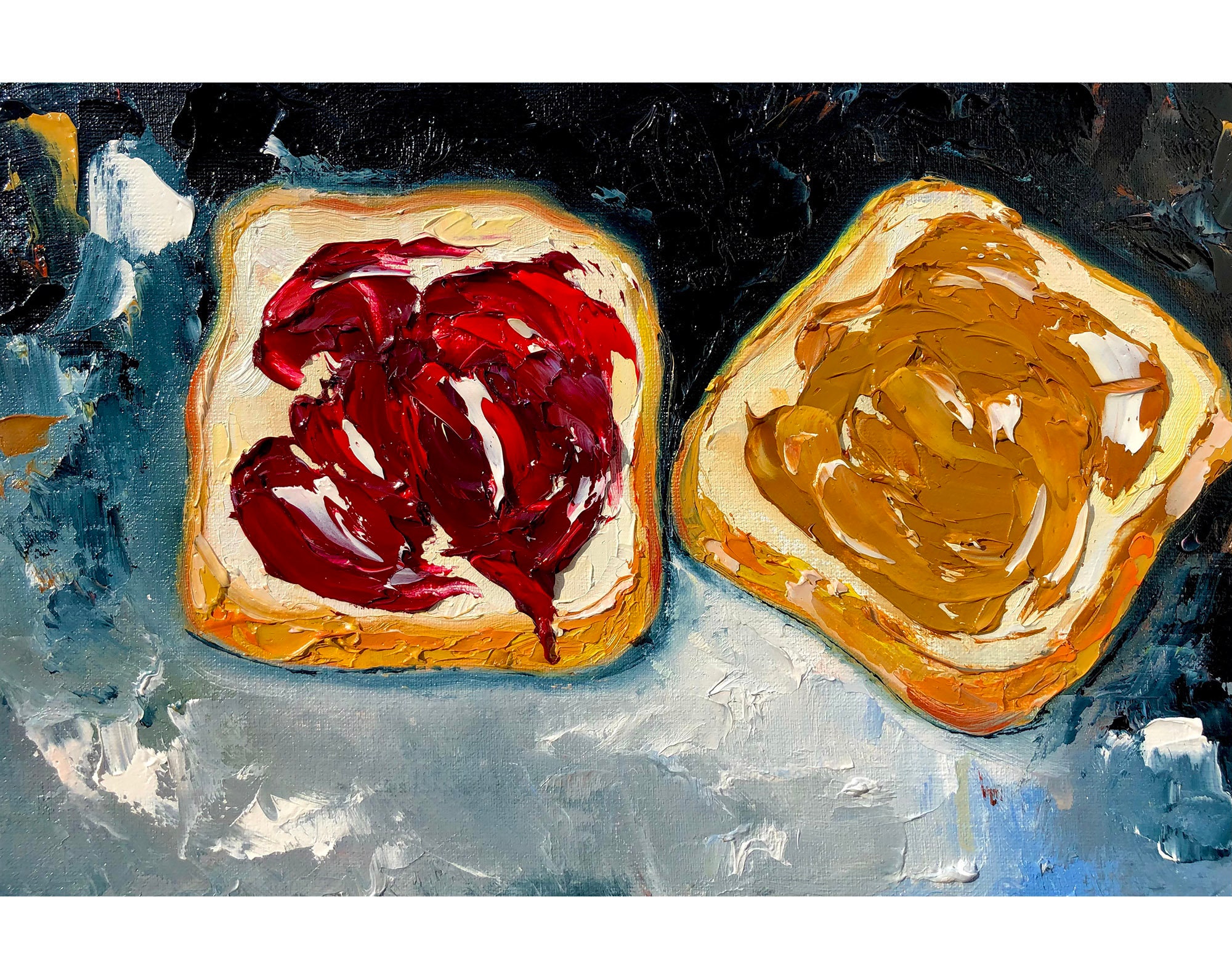This detailed painting presents an open-faced peanut butter and jelly sandwich with two slices of white bread positioned side by side. The slice on the left features a vibrant red jelly, possibly raspberry, smeared in random directions, while the slice on the right displays a smooth, brownish peanut butter, also applied haphazardly. The bread crusts are a lighter brown color, adding a touch of realism to the depiction. The overall composition is highly textured, with the background showcasing an abstract blend of black, gray-blue, and hints of orange. This uneven, slabbed-on paint enhances the three-dimensional feel of the artwork, creating a visually engaging and tactile experience.